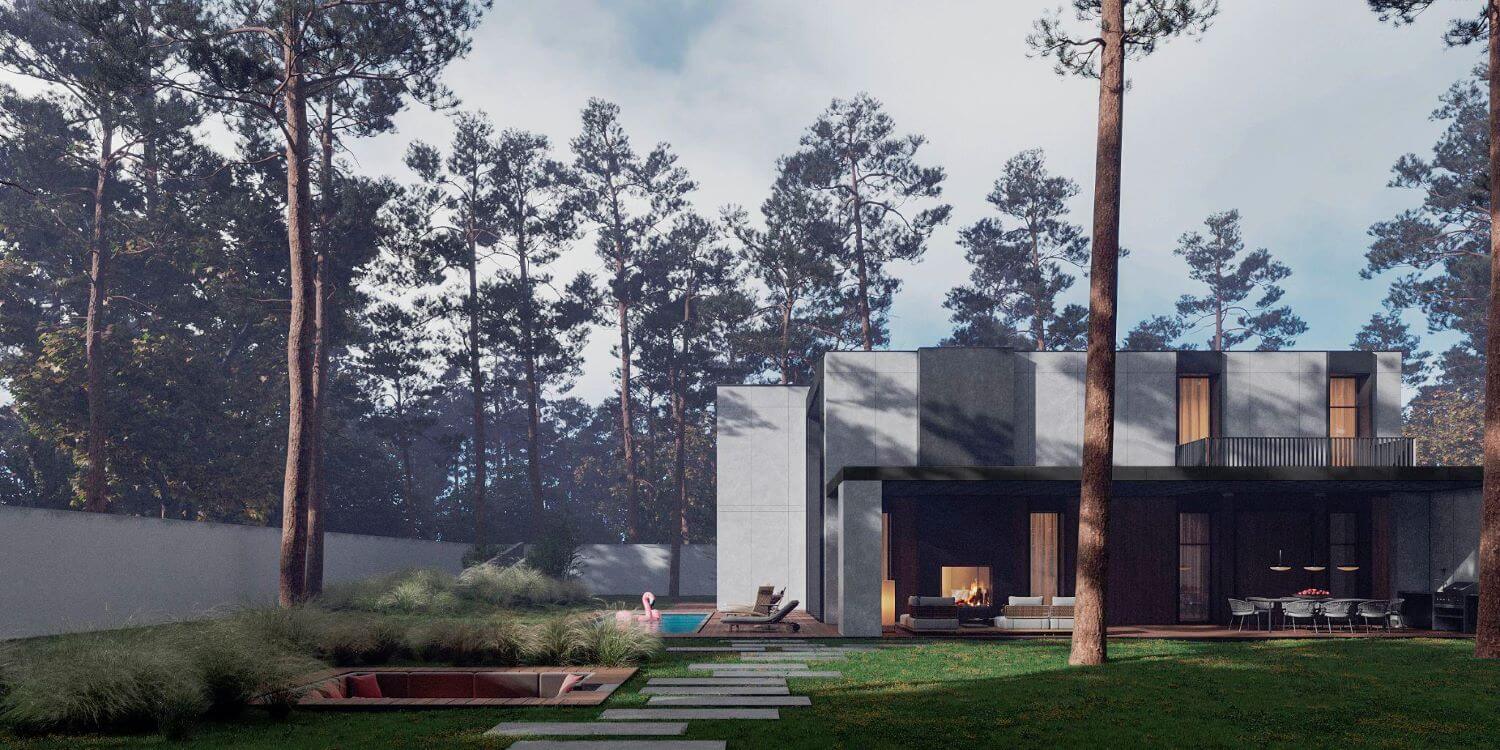The image depicts a computer-generated outdoor setting featuring a modern two-story residential house with a flat roof and a mix of brown and white exterior walls. The house is situated in the lower right-hand corner of the image. The upper level boasts a small balcony with a fenced area, while the lower level includes a spacious patio furnished with a table and chairs, and additional seating under a large awning. Near the patio, there is a fireplace on the left side.

In the foreground, a well-maintained lawn stretches across the image, bordered on the left and back by a tall white fence. Two towering pine trees stand prominently in the yard, creating a natural frame for the scene. Adjacent to these trees, a pathway made of large rectangular cement blocks leads towards the patio.

To the left of the house, there is a small in-ground hot tub area, currently without water, edged by bushy shrubs. Nearby, a small swimming pool featuring a pink flamingo float is surrounded by patio chairs, including a lounge chair. Additional details include scattered shrubs across the yard and strategically placed low-level lighting.

The sky overhead is mostly blue with patches of clouds, suggesting it is late in the day. In the background, a row of tall evergreen trees adds depth to the landscape. The house’s windows are illuminated, indicating lights are on inside. Lastly, a distinctive gray stone chimney is visible on the right edge of the building.